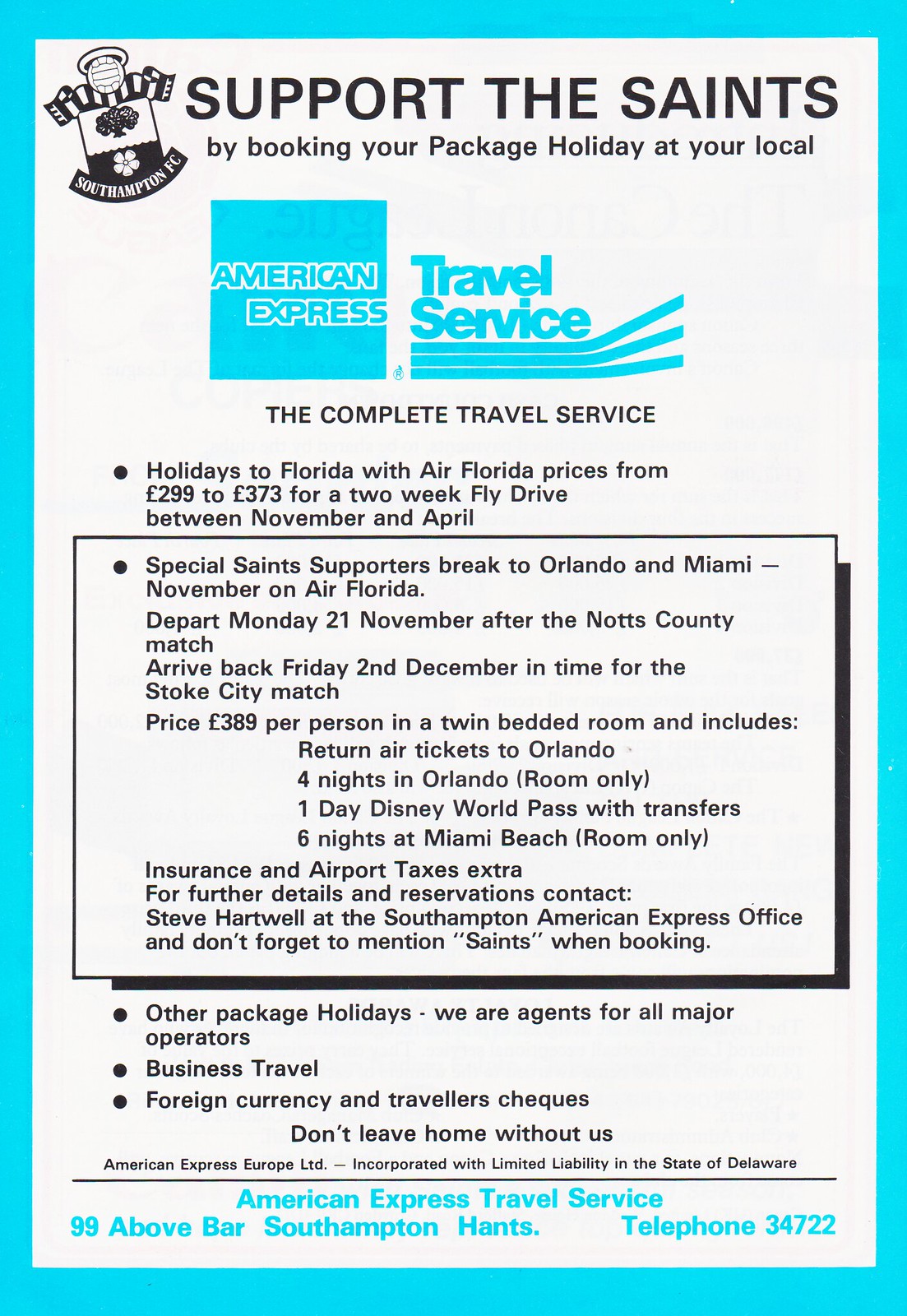Promoting unforgettable soccer fan travel experiences, this detailed advertisement features a blue-bordered design with a white background, showcasing the Southampton FC banner in the top left corner, complete with a graphic of a hat, soccer ball, tree, and flower. The bold black headline reads, "Support the Saints by booking your package holiday at your local," followed by an eye-catching blue text for American Express Travel Service. 

With an emphasis on their comprehensive travel offerings, the ad details holidays to Florida with Air Florida, featuring prices from £299 to £373 for a two-week fly drive between November and April. Highlighting a special deal, a black box announces "Special Saints Supporters Breaks to Orlando and Miami" in November for £389 per person, which includes return air tickets to Orlando, accommodations (four nights in Orlando with a room-only plan and six nights at Miami Beach with a room-only plan), a one-day Disney World pass with transfers, airport taxes, and insurance.

The ad concludes by encouraging fans to contact Stephen Hotwell at the Southampton American Express office for further details and reservations, and importantly, to mention 'Saints' when booking. At the bottom in blue text, the American Express Travel Service contact information is prominently displayed: "American Express Travel Service, 99 Above Bar, Southampton, HANTS, Telephone 34722."